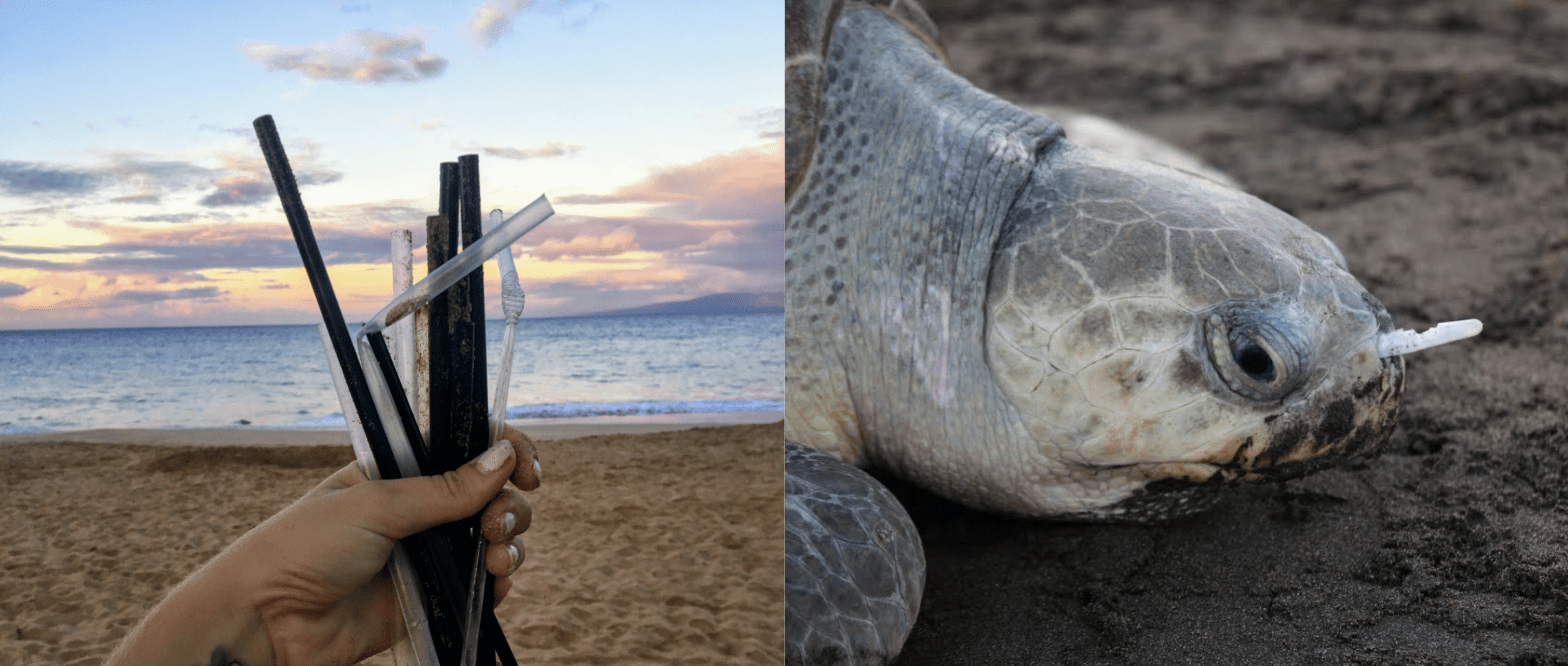The image is a powerful juxtaposition of two realities highlighting the impact of pollution on marine life. On the left, a serene beach sunset paints the backdrop with calm sea waves and a light blue sky tinged by dark clouds. A left hand with nail polish, likely a woman’s, holds a cluster of wooden sticks and plastic straws collected from the sandy shore, symbolizing both the beauty of nature and the effort to preserve it. The adjacent right image presents a close-up of a tortoise head, lying on dark sand, its gaze directed rightward. The tortoise, with its grey scaly skin and flippers visible, has a white plastic straw lodged painfully in its nostril, emphasizing the devastating effects of human negligence. Together, the side-by-side images juxtapose the hopeful act of cleanup against the heartbreaking reality of wildlife suffering, urging viewers to take responsibility for their litter.